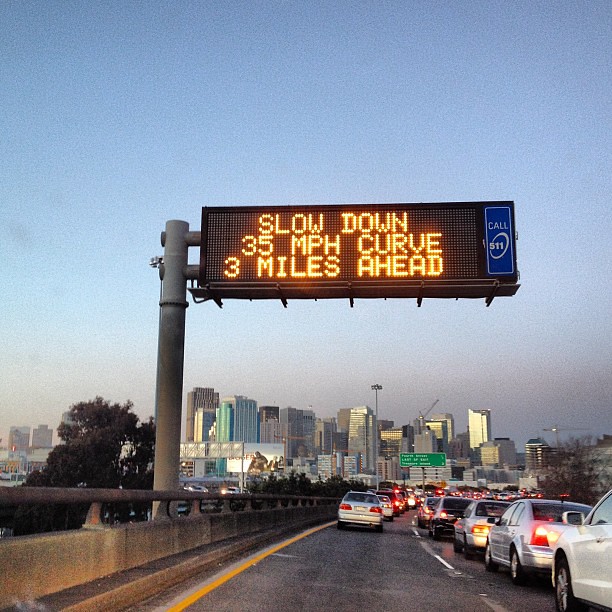This photograph, likely captured from a dash cam, depicts an elevated freeway interchange during a busy time of day with heavy traffic. The scene shows two lanes of bumper-to-bumper traffic, with most cars having their brake lights on. The road curves and merges into a larger freeway, framed by a thick cement railing and a sturdy metal rail running its length. Elevated above the landscape, the vantage point allows a partial view of tree tops below.

A prominent feature in the image is a tall metal pole on the left side, supporting a large digital traffic sign with an orange-yellow dot matrix display over a black background. The sign reads "Slow down, 35 mph curve, 3 miles ahead". Just beneath it, there's another blue sign with the text, "Call 5-1-1." A distant cityscape punctuates the background, showcasing tall apartment buildings and skyscrapers, hinting that the freeway leads toward a larger urban area.

The photograph is captured under a dimly lit sky, suggesting early morning or late afternoon, with a muted blue hue. The right lane of traffic is particularly congested, amplifying the sense of heavy traffic, while the left lane appears slightly less crowded. The detailed congestion and signages emphasize caution for drivers approaching the upcoming curve.